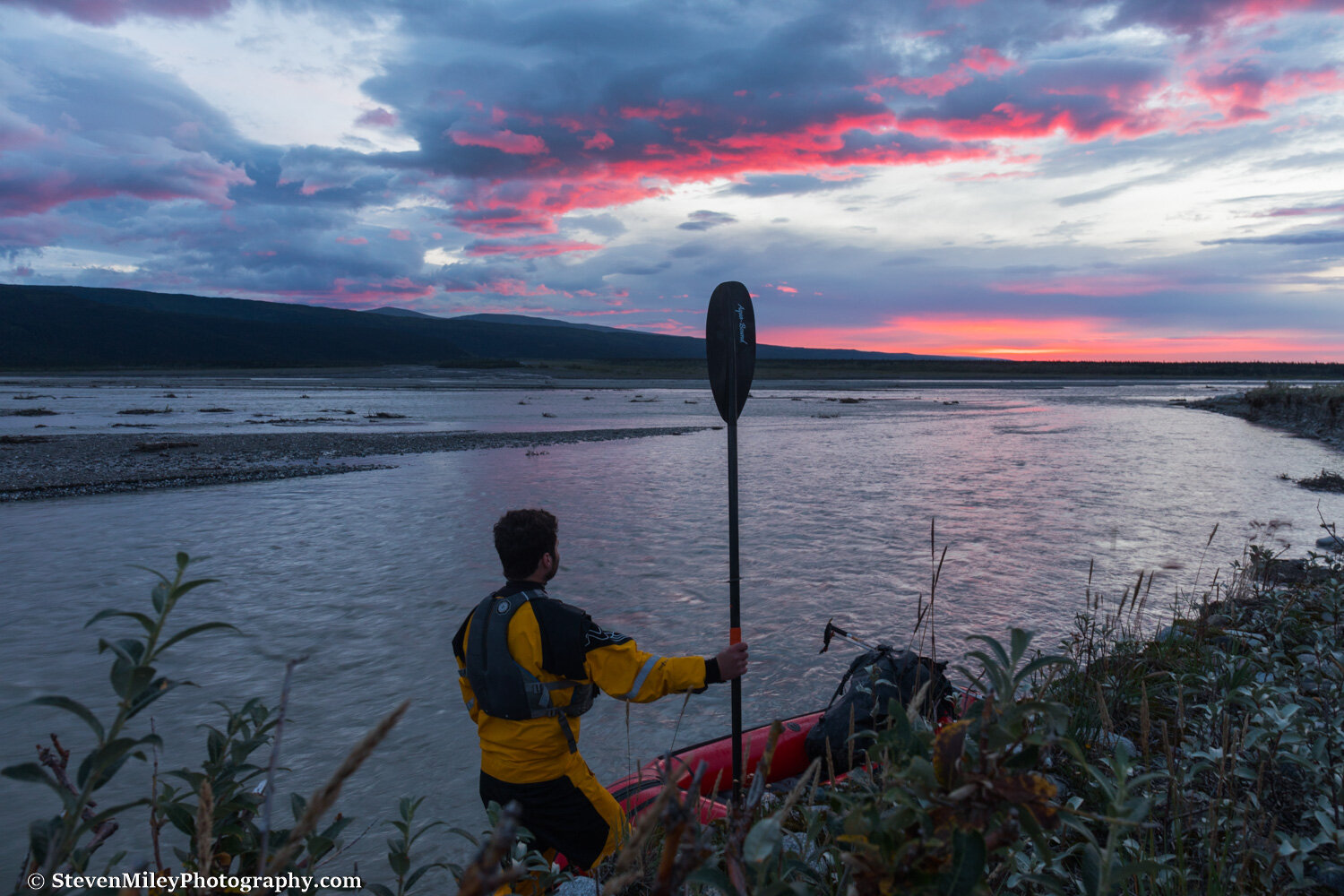The image captures a serene moment, likely during either the early morning or evening, as suggested by the sky's blend of orange, pink, and blue hues hinting at sunrise or sunset. In the foreground, a man dressed in a yellow long-sleeve top and black-and-yellow striped pants with a gray life jacket sits in a red kayak or raft positioned near the right bank of an estuary. He holds a paddle straight up in his right hand and gazes towards the expansive water and the glowing sky. The lower right corner features some obstructing grasses. Across the estuary, low hilly mountains stretch along the horizon under a cloud-mottled sky. A copyright mark in the lower left corner reads "©stevenmileyphotography.com," affirming the image's authenticity.